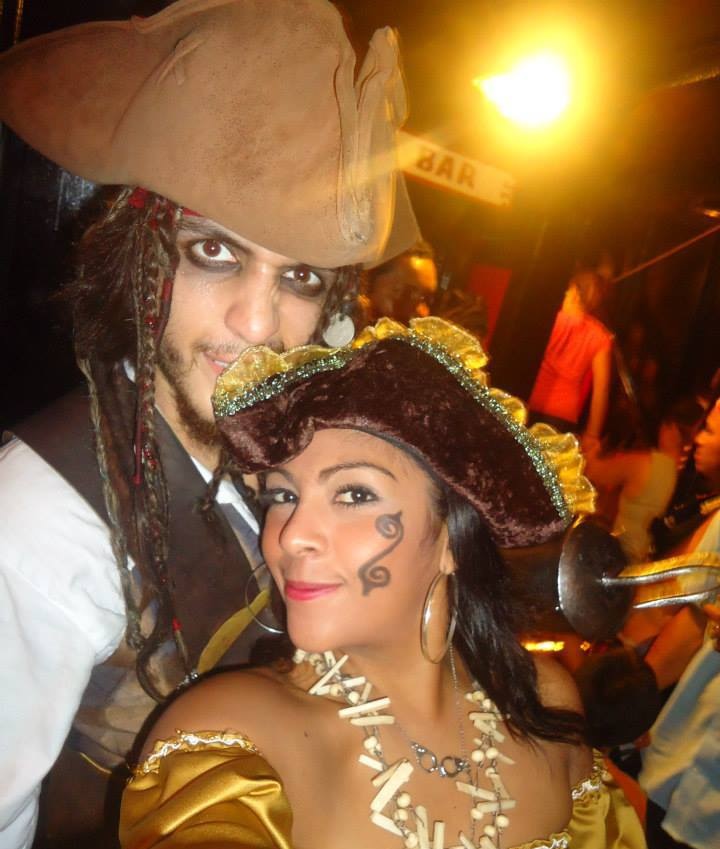In this photograph, two people are posing in costume, vividly capturing a pirate-themed event. In the foreground stands a woman adorned in a distinctive tricorn hat, lavishly decorated with sheer frills on top and golden ruffles along the edges, crafted from a rich brown felt. Her notable accessories include large silver hoop earrings and a striking fake bone necklace. Her left cheek features a playful backwards "S" marker tattoo, complementing her ensemble of a gold, shoulderless dress with subtle white trim visible at the bottom edge of the frame. Her dark brown, straight hair elegantly cascades down her back.

Behind her, to the left and partially concealed, a man channels Captain Jack Sparrow in his pirate attire. He sports a brown felt tricorn hat, framed by long dark hair tied into braids, and accented with dramatic black eye makeup. His costume includes a white shirt beneath a brown vest, completing his swashbuckling look. The close-up nature of the photograph focuses on their heads and torsos, with the background out of focus, though hints of a dimly lit room and out-of-focus figures can be discerned. A bar sign hangs diagonally on the distant wall to the right, and the scene is lit by a dim yellowish light source in the upper right corner, with an additional flash clearly illuminating the pair. This dynamic image captures the vibrant, immersive spirit of the event with a detailed portrayal of the duo's elaborate costumes.